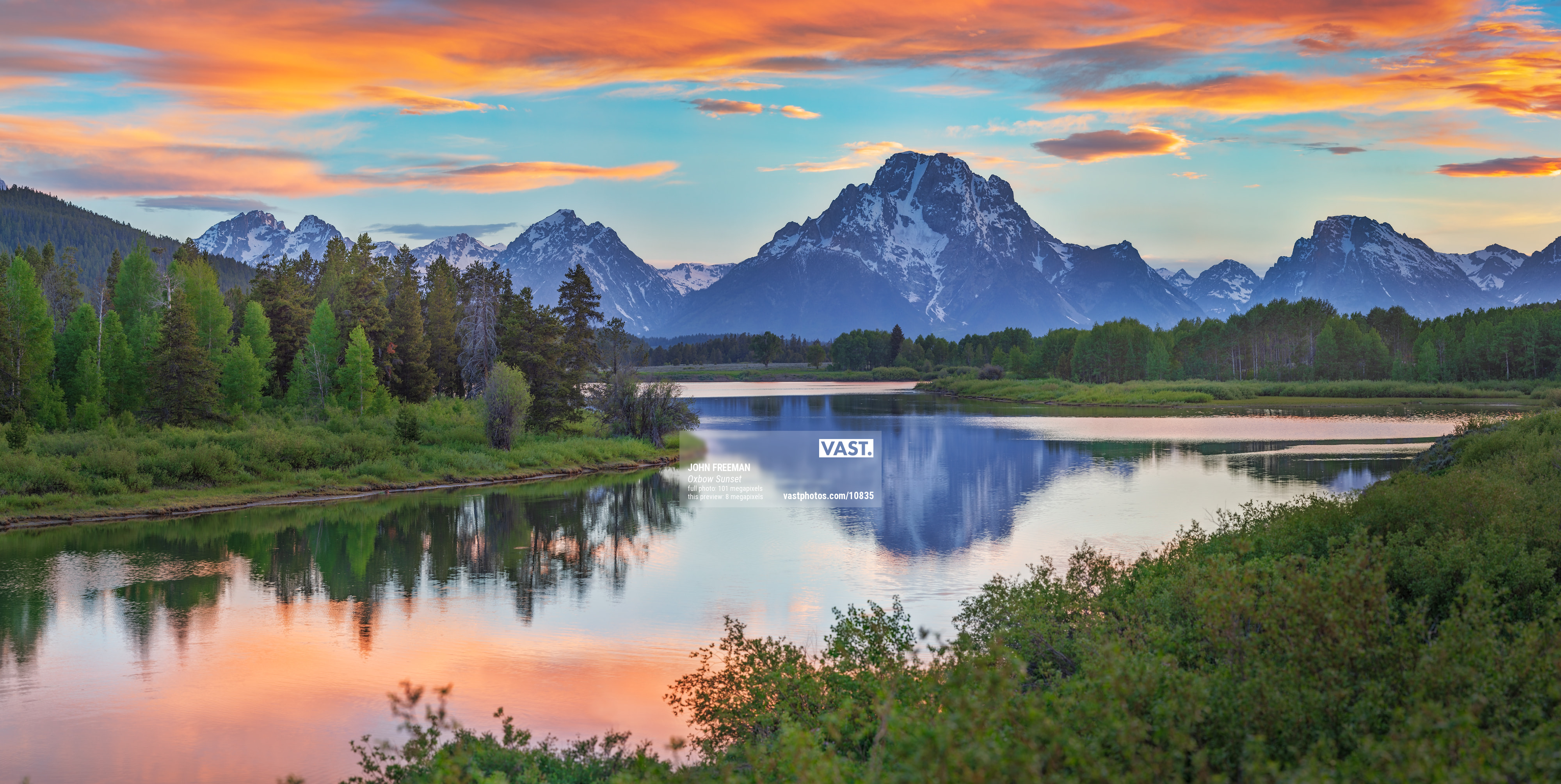This breathtaking nature photograph captures a serene mountain landscape with a calm, reflective body of water centered amidst a stunning array of natural elements. Framed by rugged, snow-capped mountains under a sky adorned with red-tinged clouds, indicative of either sunrise or sunset, the scene radiates tranquility. Dense evergreen trees populate the left side of the foreground, contrasting with a more sparse scattering of green weeds and bushes on the right. The still water, resembling a large pond or lake, mirrors the vibrant sky and jagged mountain peaks, enhancing the peaceful ambiance. Subtle digital text in the center of the image spells out "VAST," further emphasizing the expansive beauty of the scene. The photograph's vibrant color palette includes hues of orange, yellow, dark and light green, black, white, and light blue, adding to the visual richness of this outdoor setting.